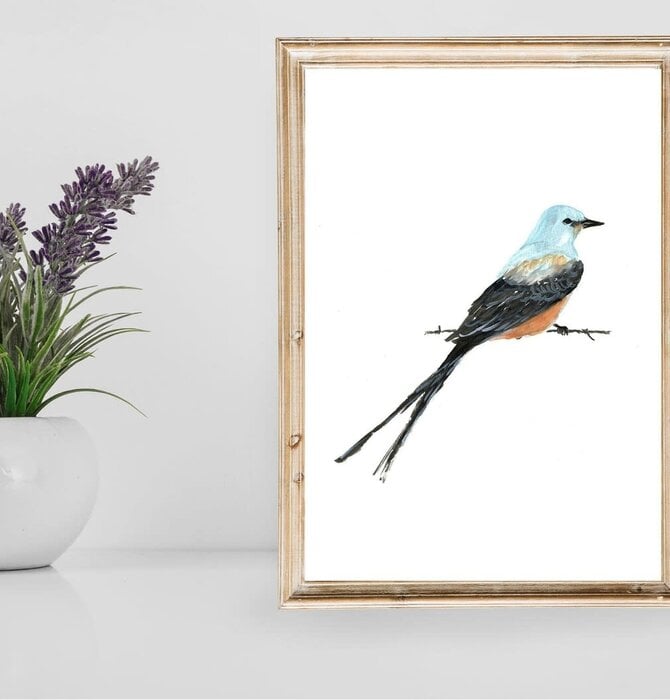The image showcases a tan-framed painting positioned on a white table against a white wall. At the center of the painting, a bird is perched on a simple, black twig. The bird features a distinctive appearance with a white head, black beak, black wings, a tangerine-colored breast, and an impressive tail composed of long dark feathers with a white center. To the left of the painting, there is a dish-like vase with a live plant. The plant has tall stems adorned with elongated light purple flowers and green leaves, extending slightly towards the right. The entire scene is minimalistic and serene, with a harmonious blend of neutral and natural tones.